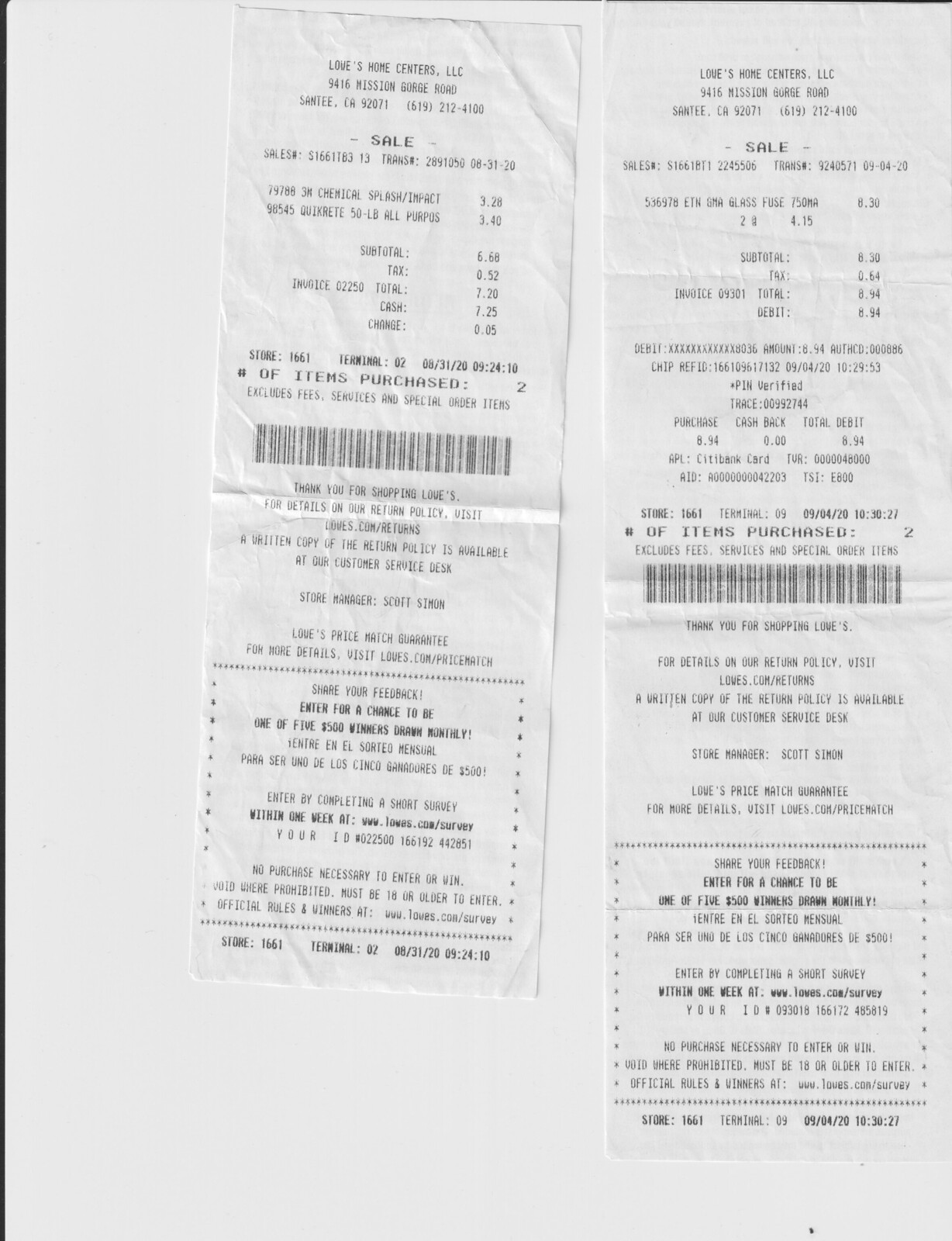This image features two white paper receipts laid side by side on a white surface, possibly a table, with a black border visible at the edges of the image. Both receipts are from Lowe's Home Centers LLC, located at 9416 Mission Gorge Road, Santa Fe, California 92071. The phone number is listed next to the address on the right-hand side of the receipts. The receipt on the right is longer than the one on the left. Each receipt indicates a different date: one from August 31, 2020, and the other from January 4, 2020. Both receipts note the purchase of two items. The first receipt has a subtotal of less than $5, suggesting small or discounted items, and mentions a chemical splash purchase among its details. The second receipt records a purchase amounting to around $4.30. The image focuses solely on these receipts without any additional context or surrounding items.